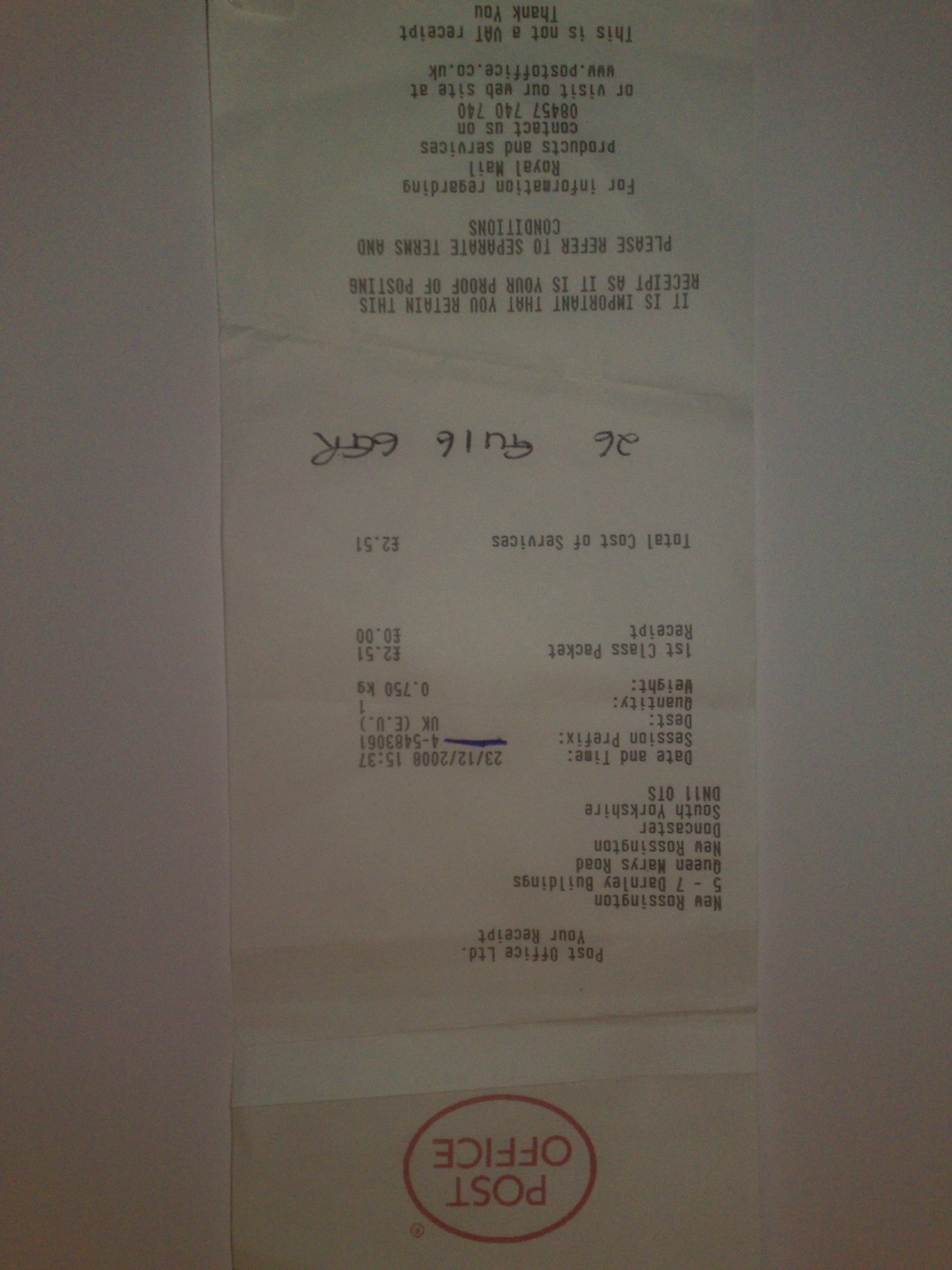The photograph features an upside-down receipt placed on a white surface, making the text challenging to decipher. The top of the receipt, which appears at the bottom of the image due to its orientation, is marked with a red circle containing the words "post office" in red letters. Printed on the receipt are several blocks of text detailing quantities, weights, and prices of items, including what seems to be a total amount of £12.51. Handwritten numbers, starting with "26," are visible below this total. A prominent crease runs through the receipt, adding to the difficulty in reading the details. At the very bottom, which appears at the top due to the upside-down orientation, the receipt says "thank you" and includes a phone number.